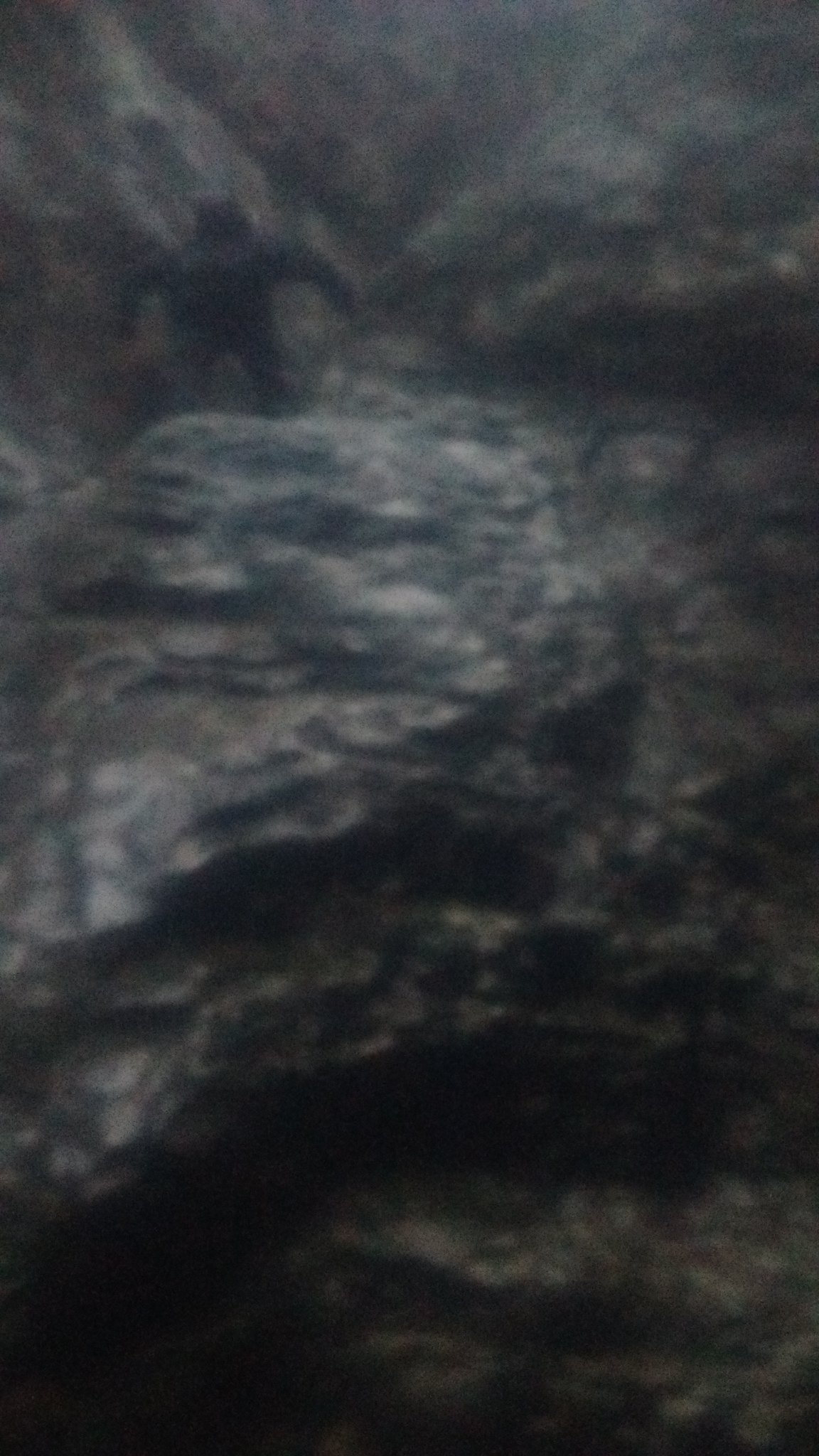The image appears to be a somewhat blurry and grainy depiction of a steep, craggy rock face, possibly computer-generated or from a video game, rather than a photograph. The rocks are large, boulder-like formations characterized by a mix of granite gray and white hues, interspersed with very dark, black shaded areas, particularly at the bottom of the image. There are small ledges and outcrops on the rock where climbing would be technically possible. Dominating the scene is a mysterious figure with spread-apart legs and outstretched arms, perched on one of the prominent outcrops. This figure, which could be interpreted as either a bear-like creature, a person in a bear costume, or some other fantastical entity, adds an element of intrigue to the rocky landscape. The lack of visible sky or ground and the overall low resolution and focused details on the rock textures contribute to the enigmatic and somewhat surreal quality of the image.